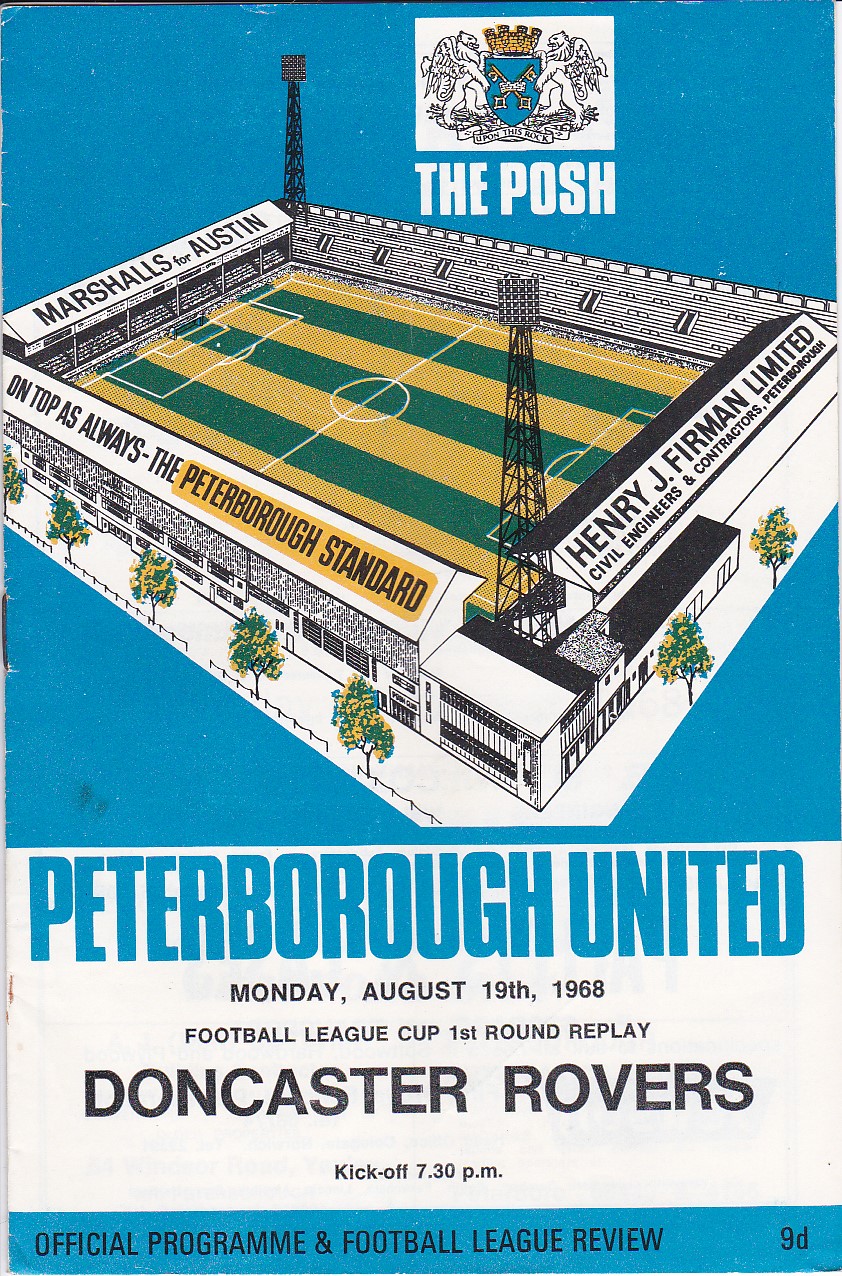This image is a highly detailed cover of a commemorative program for a British football match, likely for the Peterborough United soccer team. Dominating the cover is an intricate illustration of a soccer stadium with gold and green stripes marking the field, complete with a center circle, half-field mark, and white outlines around the goals. The background is blue, adding a striking contrast. Text adorning the stadium's roof includes advertisements: "Marshals for Austin" and "Henry J. Furman Limited, Civil Engineers, Contractors, Peterborough." Another inscription reads, "On top as always, the Peterborough Standard."

Prominently featured on the cover is the team's heraldic logo, consisting of two winged lions holding a coat of arms with two crossed keys and a gold crown that resembles battlements. The text "Vipash" and "The Posh" appear nearby, referring to the team’s nickname.

Additional information at the bottom of the program details a specific match on Monday, August 19th, 1968, part of the Football League Cup's first-round replay against Doncaster Rovers, with kickoff scheduled for 7:30 p.m. The program is marked as the official program and includes a "Football League Review," all priced at 9-D.